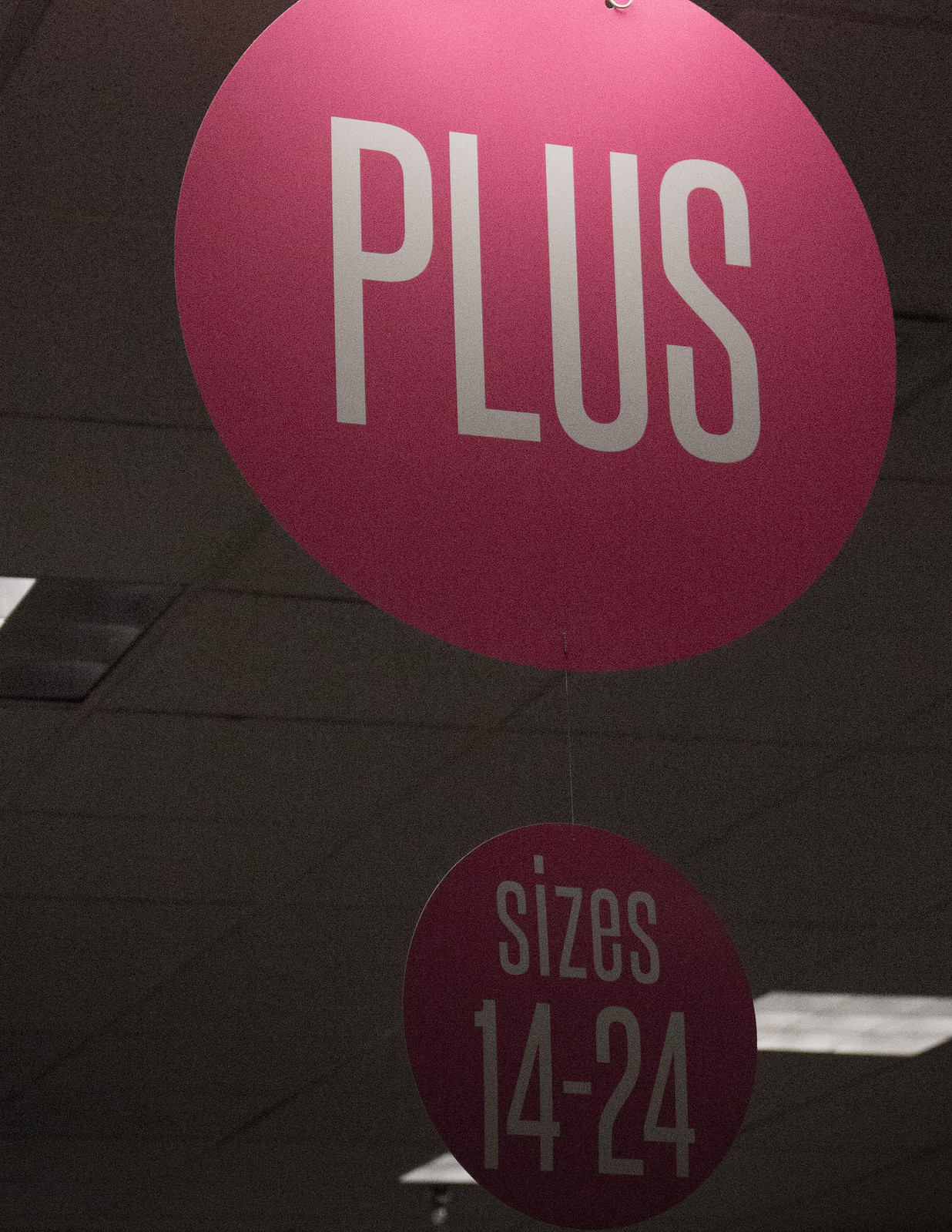The image showcases two vertically aligned, circular signs set against a commercial ceiling backdrop. The upper sign is larger, featuring the word "PLUS" in bold white letters centered on a vibrant pink background. Directly below it, a smaller circular sign displays the text "size 14-24" in similar white lettering. The background reveals a white ceiling with a grid-like pattern and integrated lighting fixtures, suggesting an indoor retail environment.